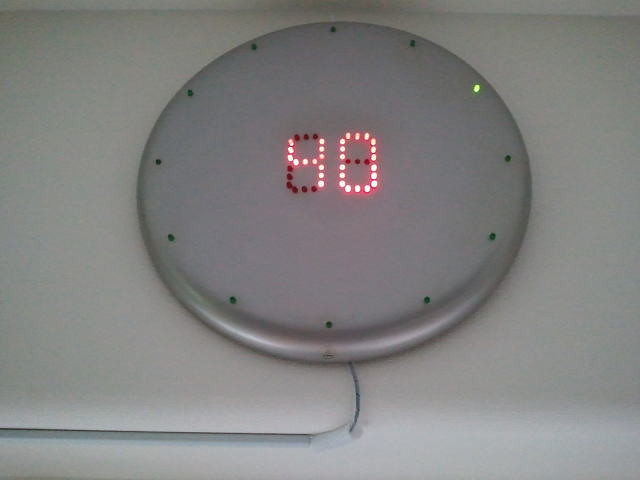This up-close image showcases a unique and modern digital clock mounted high on a white wall, just below the white ceiling. The clock, resembling a silver disc or metal frisbee, is circular with rounded edges and a flat top, giving it a sleek, contemporary look. Around its outer edge, a series of small light diodes act as markers, with one diode illuminated green at the two o’clock position. At the center of the clock, tiny digital diodes form the number "40" in red, indicating the current minute. The remaining diodes are unlit but are designed to create various numbers as needed. A thin, off-white wire extends from the bottom of the clock, encased in a neat, very thin metal or plastic cover, adding to the organized aesthetic. This clock not only tells time but also stands out as a modern decorative piece against the pristine white backdrop of the wall and ceiling.